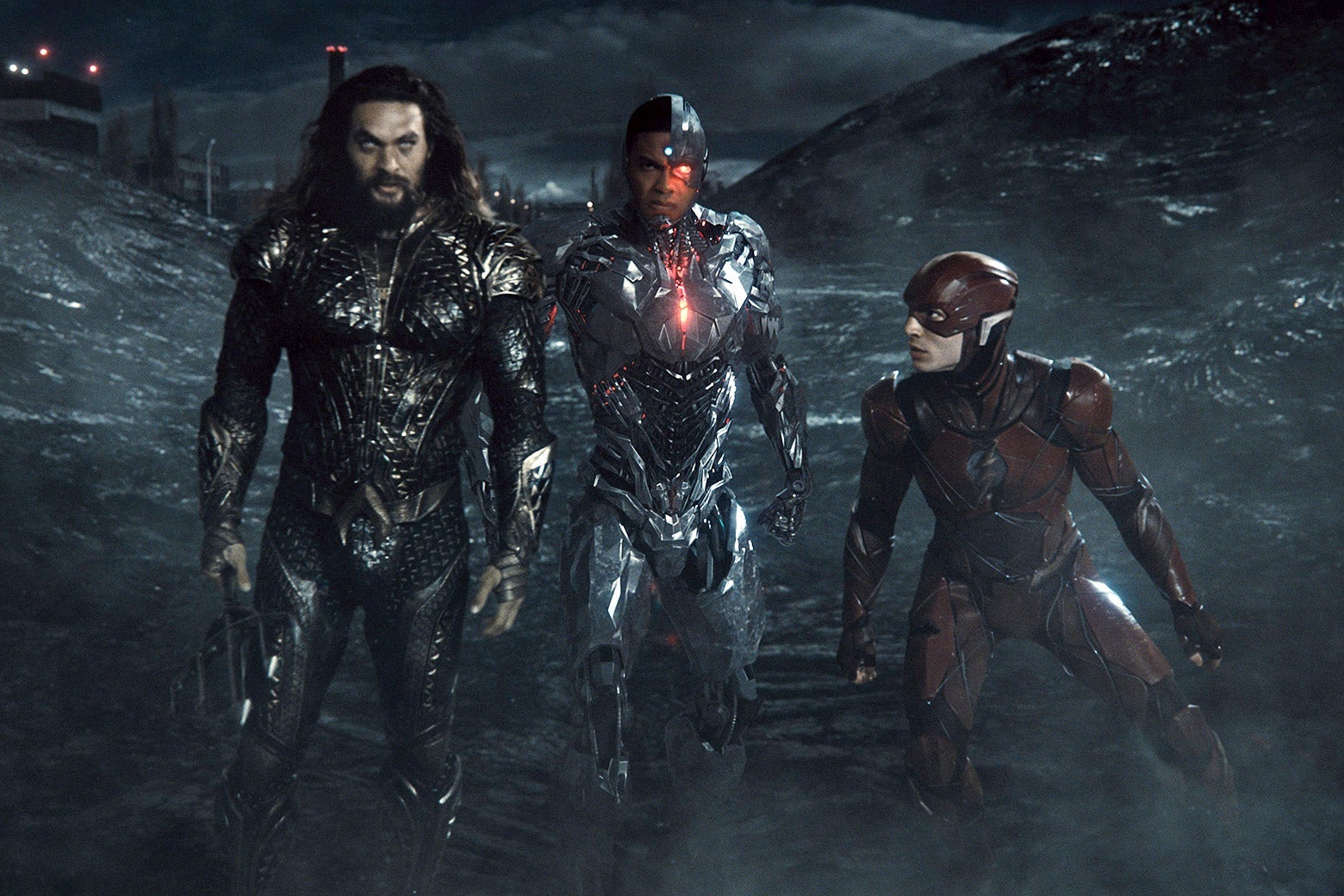The photo captures a dramatic, nighttime scene with three iconic DC superheroes standing poised for battle against a dark, ominous backdrop. On the left stands Aquaman, his long dark brown hair flowing over a gold, fish-scale-textured armor that glistens under the ambient light. In the center is Cyborg, a formidable figure with a fully mechanized, metallic body featuring a red light over one eye, emphasizing his robotic nature. On the right, the Flash, adorned in a deep red suit, crouches slightly below his comrades, exuding readiness and speed. Behind them, a massive wave of water rises, highlighted by the gray and black hues that shimmer, creating a stark contrast to the faintly illuminated cityscape beyond. This image not only captures the superheroes' readiness for action but also conveys the depth and intensity of their environment.